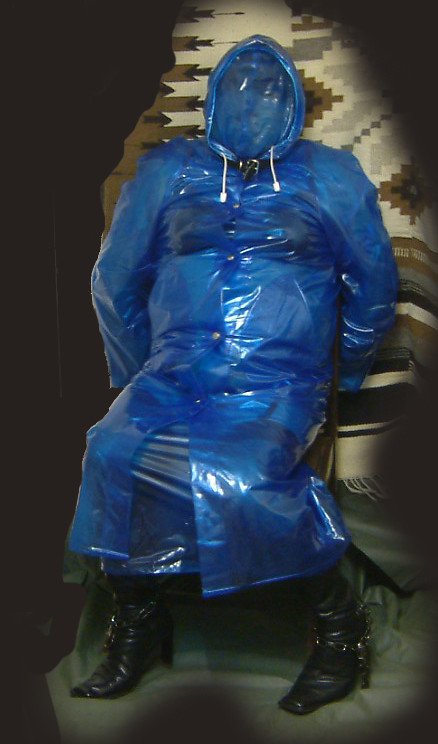The photograph depicts a person seated in a brown wooden chair, wearing a transparent blue raincoat that extends down to their legs. Underneath the raincoat, they don black stockings with garter belts, providing a glimpse of their undergarments including a black bra. The individual also sports high, thin-heeled black leather boots adorned with chains around the ankles. Their face is covered by a blue mask, adding a mysterious aspect to the ensemble. Positioned behind them is a textured background of a brown, gray, and white patterned blanket with frayed strings along the edges. Despite the overall dark ambiance, the intricate details of the boots, raincoat, and fabric backdrop underscore the image, suggesting it may be a deliberate and artistic composition.